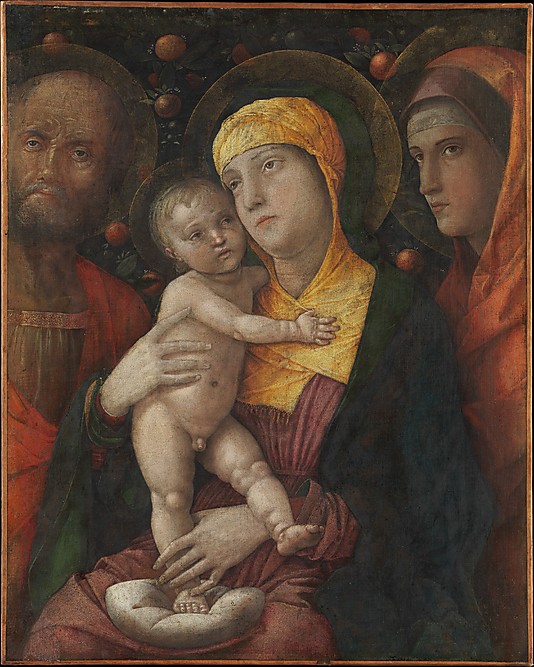This vertically oriented photograph features a captivating, ethereal Renaissance-style painting with a predominantly dark background that adds a mystical aura. At the center, there is a prominent woman, possibly Mother Mary, cradling a nude baby boy. The woman, depicted with pale skin, wears a yellow headscarf or turban, a red dress, and a dark cloak around her shoulders. The golden, semi-transparent halo behind her head, along with a similar one behind the infant, suggests their saintly status. The baby extends one leg over a white cushion on her lap while pressing his hand against her neck, and her hand cradles his chest, their heads tilted towards the left.

To the left, an older man with a beard and mustache, possibly in a brown shirt and red cloak, also bears a golden halo. He gazes outward, adding to the painting’s contemplative atmosphere. On the right, another woman adorned in a dark brown and orange headscarf, wrapped around her body like a sarong, looks slightly to her right, contributing to the composition’s sense of serene watchfulness.

The background subtly suggests a cosmic scene with floating planet-like spheres, and the entire image is framed by an ornate, gold gilt edge, enhancing its timeless, sacred quality.